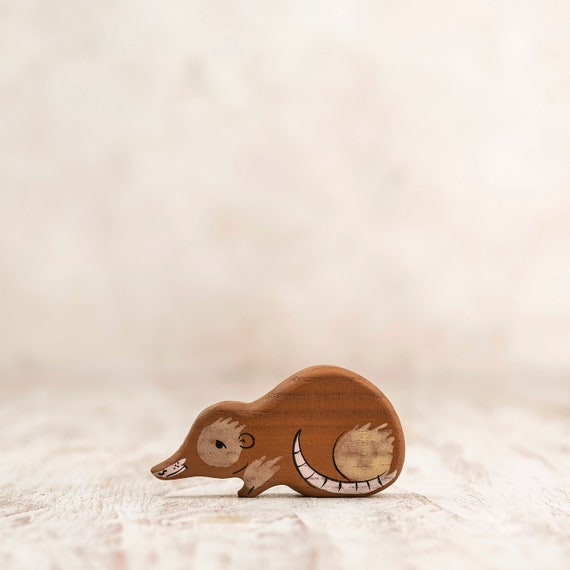In this detailed color photograph, we see a small wooden figurine of a rodent, possibly a mouse or a possum, positioned on a white wooden background. The figurine is a simple, homemade carving with a basic paint job—brown in color with minimal detailing. The pink tail is merely painted onto the wood. The creature stands upright on its feet, facing to the left, with visible features including its eye and leg. The overall appearance is plain and unembellished, reflecting a rustic and handcrafted aesthetic.